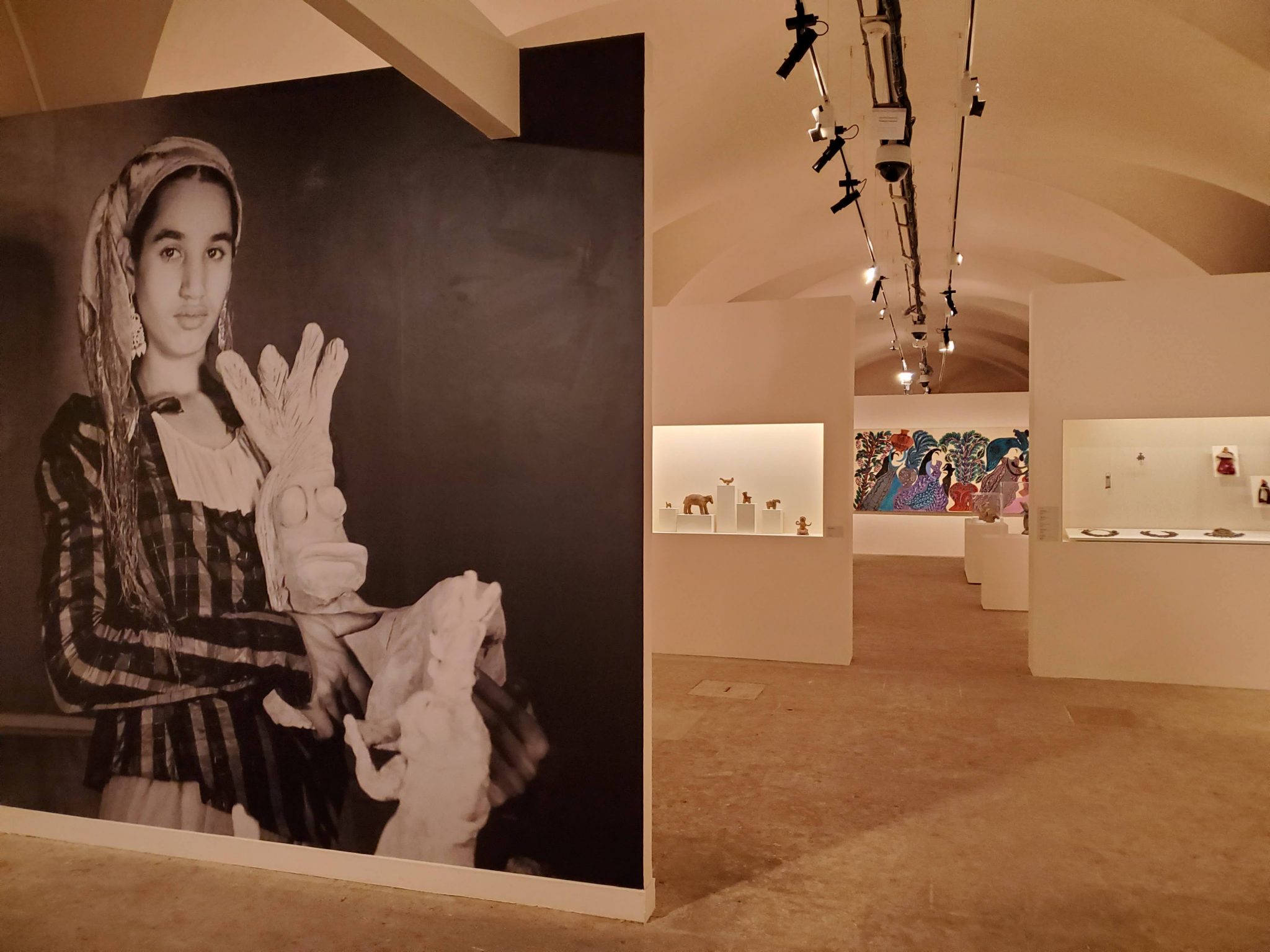The photograph captures an indoor art installation within a half-cylinder shaped hallway. The space is enveloped in a uniform tan color scheme, with matching walls, ceiling, and floor. The centerpiece of the display is a large, black and white photograph occupying an entire wall. This photograph features a woman, possibly of Navajo or Native American descent, adorned in a headscarf and a striped, pioneer-style blouse. She wears white gloves and holds a striking white stone sculpture depicting a Native American chief, characterized by pronounced facial features, including large eyes and a sizable mouth.

The photograph is part of a series of art pieces displayed on large boards or half-walls along the hallway. In the distance, a large white wall showcases a vibrant, colorful art piece dominated by hues of blue, orange, purple, and red. The installation is illuminated by track lighting affixed along the curvature of the ceiling, enhancing the visual appeal of the artworks and the overall ambiance of the space.